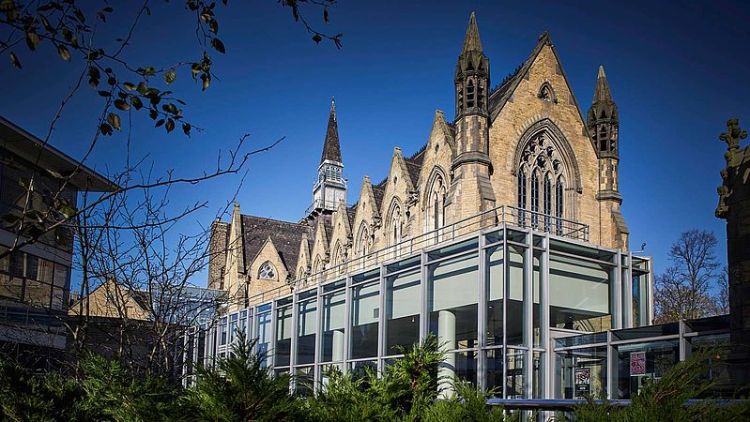This photograph showcases a striking architectural juxtaposition against a vivid blue sky. At the center stands a large, imposing building that exudes a blend of Victorian and older cathedral styles, marked by brown stone blocks and towering spires. The upper section suggests an antiquated church or cathedral, dating possibly from the 17th to 18th century, with tall steeples and stone pillars. In contrast, the lower section appears to be a modern glass and metal structure, potentially serving as an entryway or annex to the historic part.

Framing the scene, green foliage and sparse trees with bare branches are visible in the foreground. The left side of the image includes a separate, modern-looking building, partially visible alongside the natural elements. The photograph is taken from a low angle, emphasizing the height of the main building and adding depth to the composition, which seamlessly integrates the historical and contemporary architectural elements. The overall ambiance is serene and uncrowded, enhanced by the clarity of the sky and natural light.